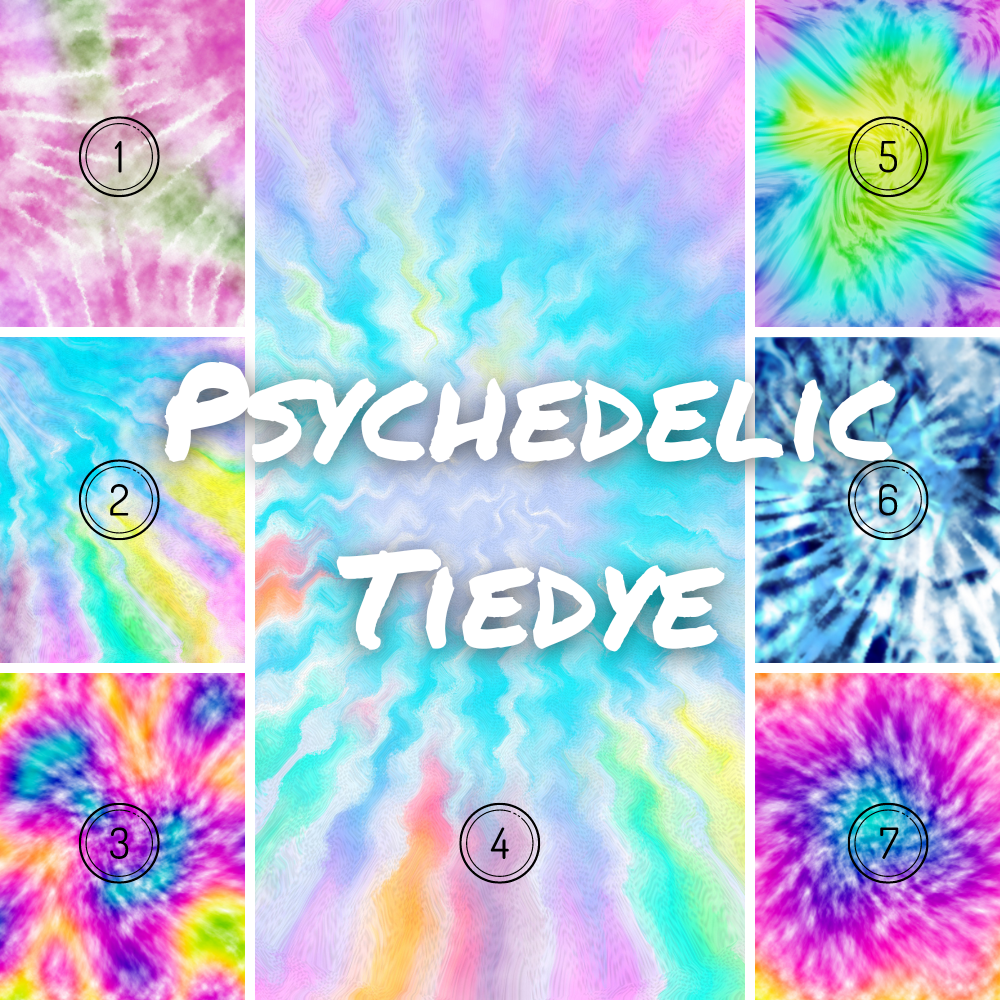The image is a vibrant, colorful display featuring multiple psychedelic tie-dye designs. Dominating the center is a large vertically oriented rectangle filled with an array of pastel colors radiating from a light lavender core. These colors include yellow, green, purple, orange, and various shades of blue, with the word "PSYCHEDELIC" in bold white capital letters prominently displayed, followed by "TIE-DYE" and the label "4" beneath it.

On either side of this central pane are three smaller rectangular sections, making a total of six additional panels arranged in a 3x3 grid. Each section exhibits a unique tie-dye pattern and is individually numbered from 1 to 7, starting at the top-left corner. The designs in each panel vary, showcasing different color combinations: Panel 1 has pink and green hues, Panel 2 features a blend of blue, yellow, green, and purple, Panel 3 combines pinks, purples, and oranges, Panel 5 includes greens, whites, and yellows, Panel 6 displays a blue and white palette, and Panel 7 is characterized by a mix of pinks and blues. The bottom right section heavily features pink, purple, blue, and yellow tones. 

This image appears to be a showcase of different tie-dye patterns, possibly for a website offering these psychedelic designs on various products.